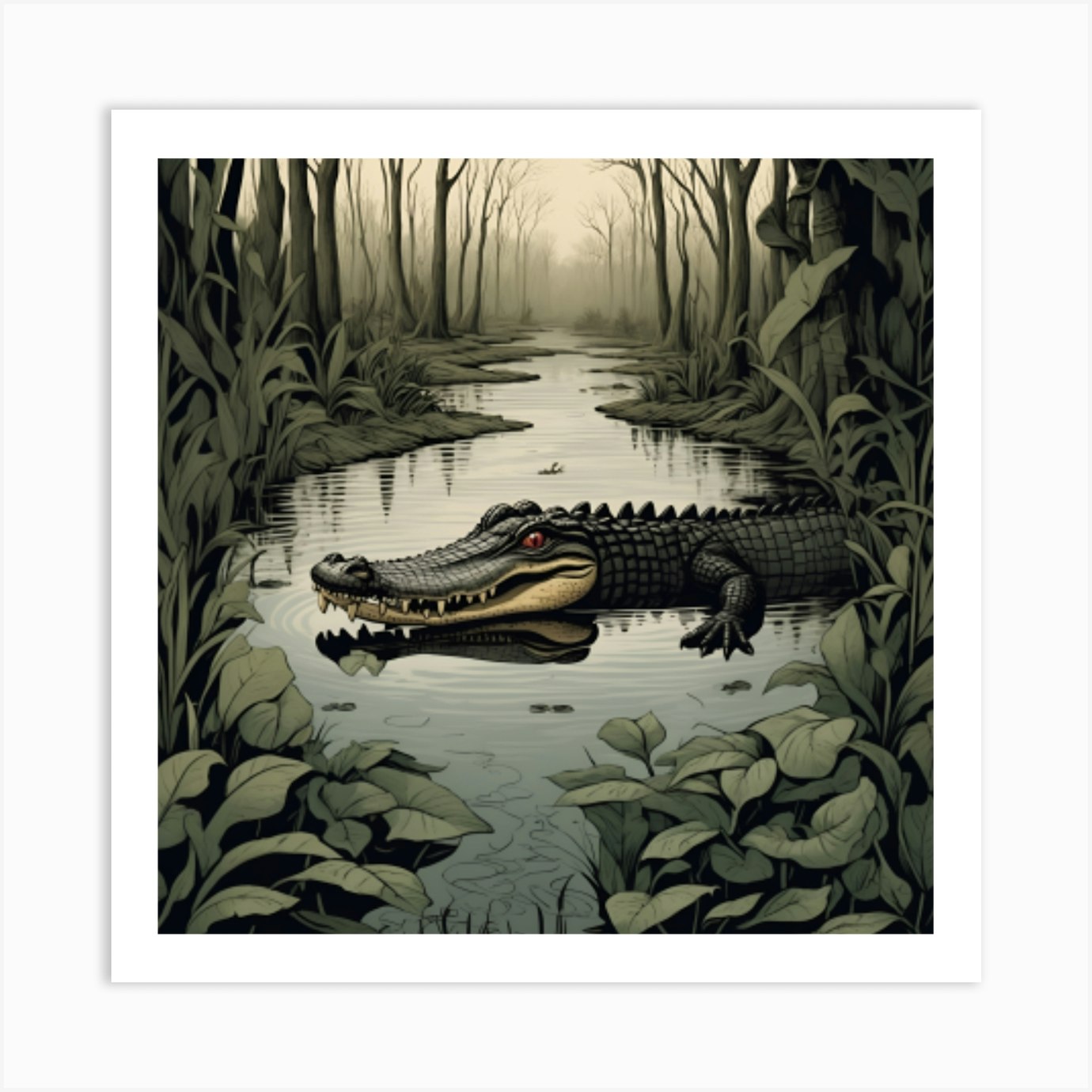The image is a computer-generated illustration depicting a swampy scene bathed in greenish hues. At the center lies an alligator, its scales characteristically rugged and mouth closed, emerging from the murky, shimmered waters surrounded by lily pads and heart-shaped weeds. This tranquil body of water is peppered with waterborne leaves, creating a lush, textured foreground. The alligator's red eyes give it a somewhat eerie look, contrasting with the otherwise muted tones of its black and light green skin. The scene extends into a foggy, white sky with barren trees in the background, enhancing the misty, mysterious atmosphere. The alligator, with an almost mischievous expression and visible sharp teeth on the top of its mouth, appears to be looking off to the side, contributing to the enigmatic charm of this swampy tableau.